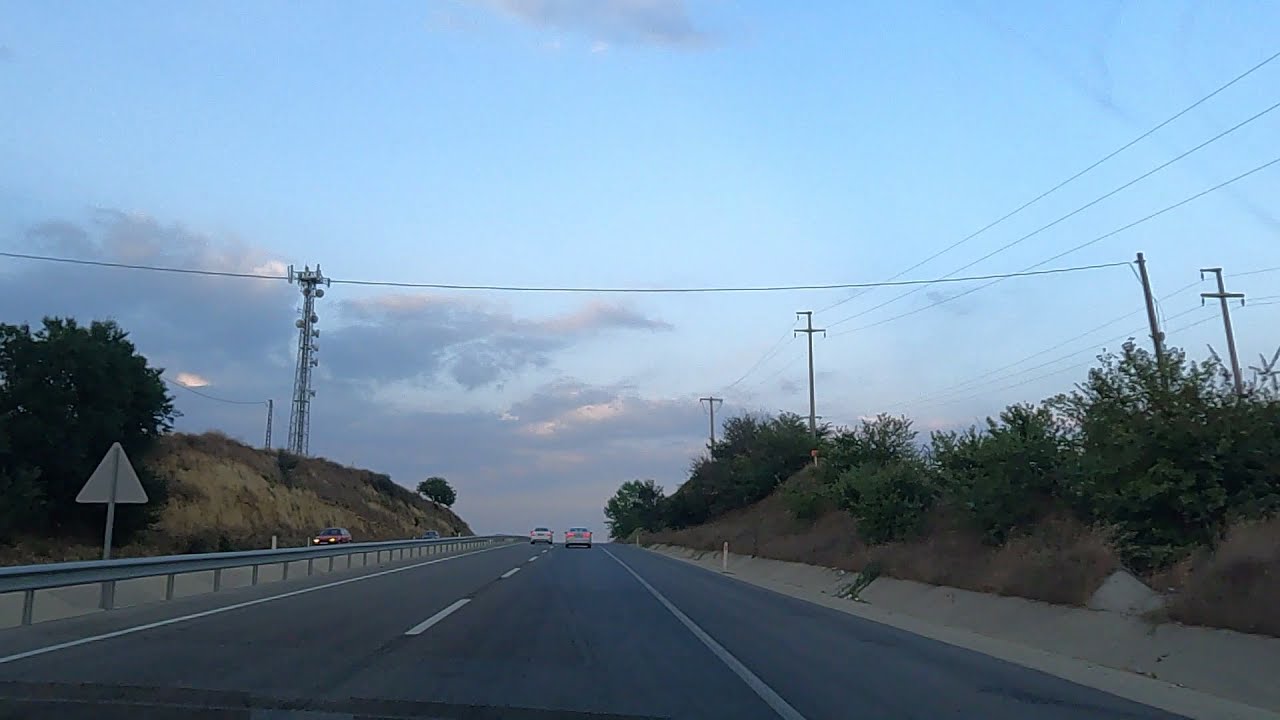The image depicts a four-lane highway from the perspective of a driver heading north. The road consists of two lanes in each direction, separated by a barrier. Two cars are visible in the lanes ahead, moving in the same direction as the viewer, while two cars travel in the opposite direction in the other set of lanes. Surrounding the highway are dry grass and green bushes, with electric poles and overhead wiring running alongside the road. A rocky area is noticeable on the right side, and there appears to be a cell tower on the left. The sky is blue with a few clouds, tinged with orange hues, suggesting it's early evening. The overall setting includes a mix of natural elements and infrastructure, creating a balanced yet dynamic roadside scene.